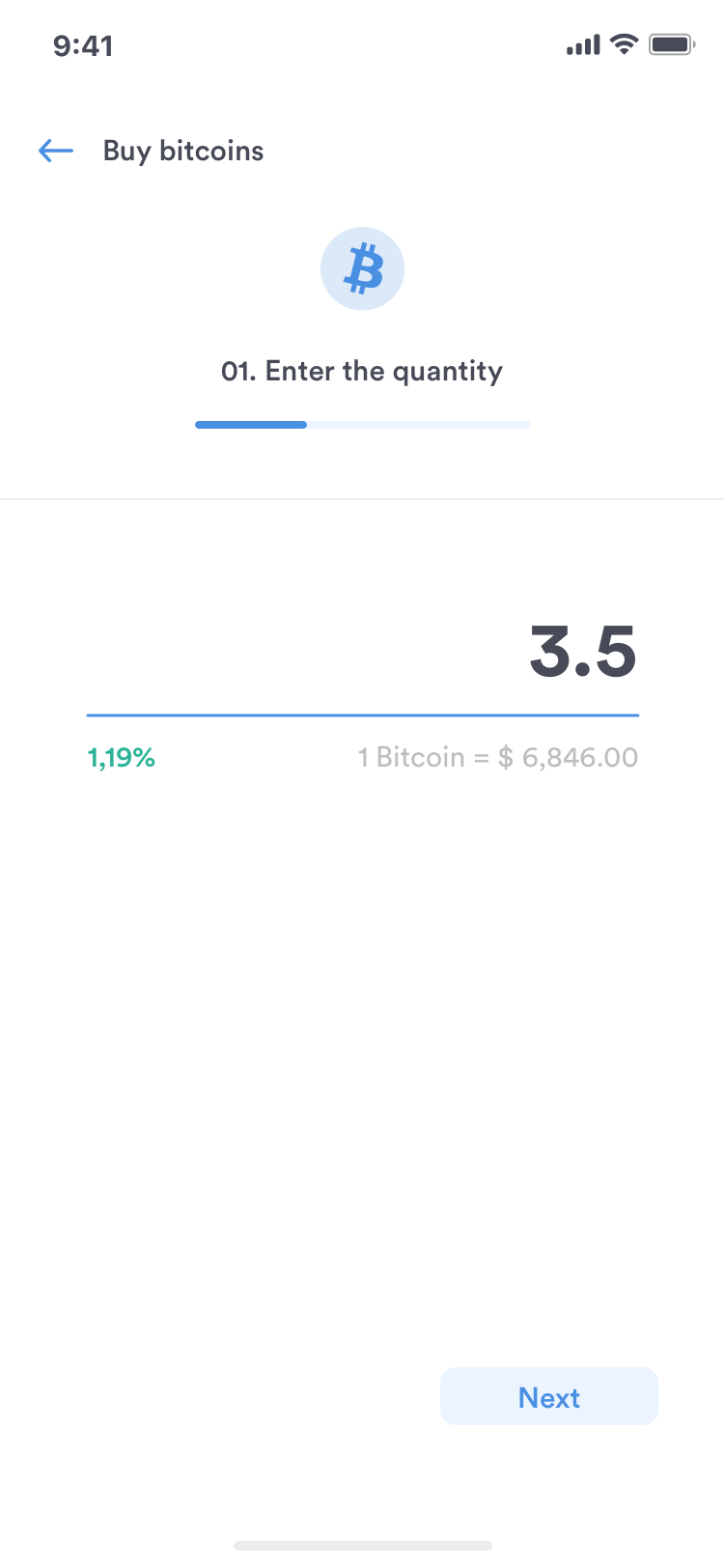Screenshot Caption: 

The screenshot features a clean, white background. In the upper left-hand corner, the time is displayed in black as "9:41". Next to it, the signal reception bars are fully black, indicating strong reception, and the Wi-Fi symbol is similarly filled, showing excellent Wi-Fi connectivity. The battery icon is almost full, suggesting a high charge level.

Below the status bar, there is a blue arrow pointing to the left, and adjacent to it in black text, it reads "Buy Bitcoin". Further down, there's a light blue Bitcoin symbol with a slightly darker blue "B" within the circle, differing from the usual orange and white color scheme.

Underneath, a prompt states "Enter the quantity" in black text, accompanied by a grey underline. To the right, in black text, it shows "3.5" with a blue underline beneath it.

On the left side in green, it reads "1, 19%," and across from it in gray, it states "1 Bitcoin = $6,846.00".

At the bottom right corner of the screen, there is a light blue rectangle with darker blue text that says "Next".